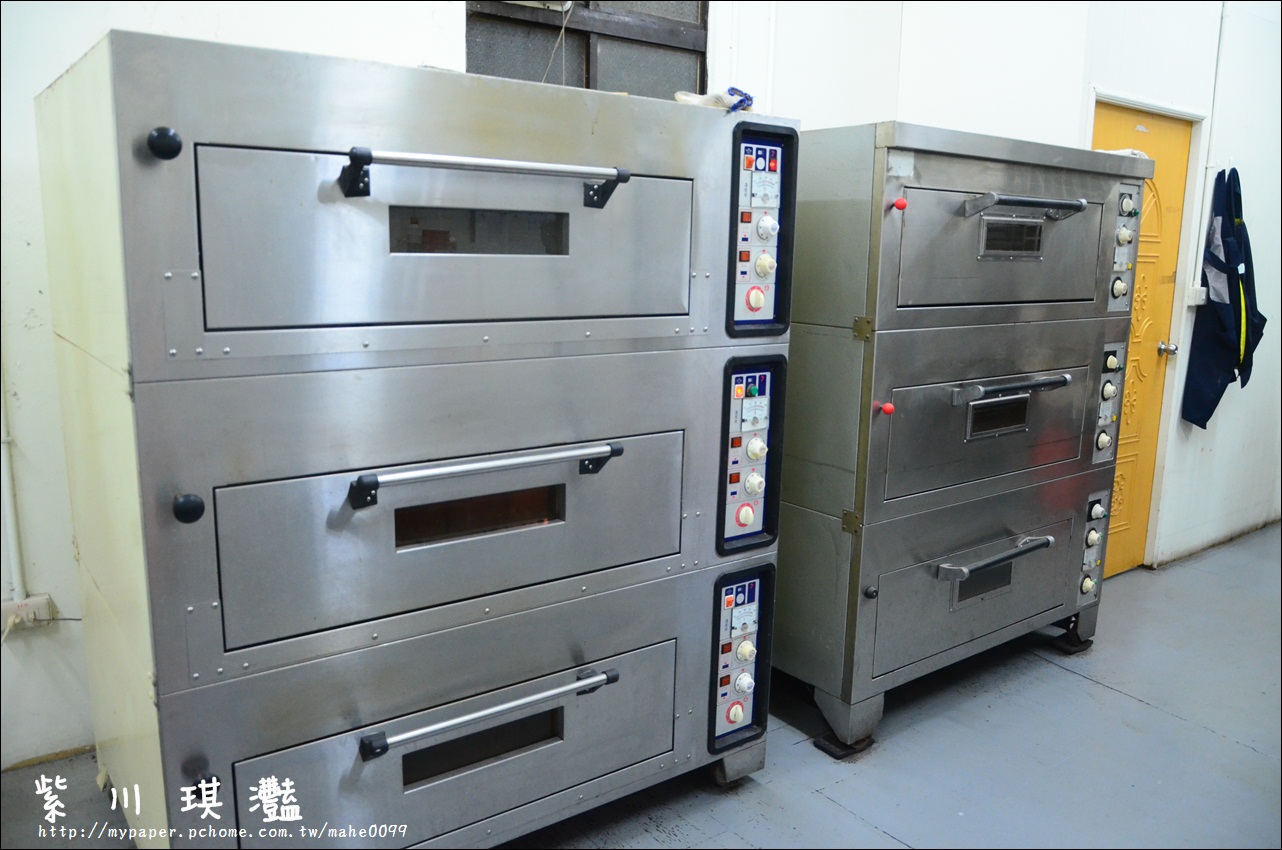The image, slightly wider than it is tall, depicts a section of a commercial kitchen. Dominating the scene are two tall, rectangular industrial ovens, each consisting of three stacked compartments. These ovens are silver with black sides and feature long silver handles on the front of each compartment, making them appear as drawers. Each oven unit is accompanied by a detailed control panel on its right, boasting a variety of white dials, red switches, and a few green ones, indicating sophisticated control mechanisms. The controls of one oven seem more modern compared to the other. To the right of the ovens stands a brown door against an off-white wall, with a black jacket hanging nearby. The lower left corner of the image includes four Asian characters, likely Chinese or Japanese, overlaid on the picture with a URL beneath them.